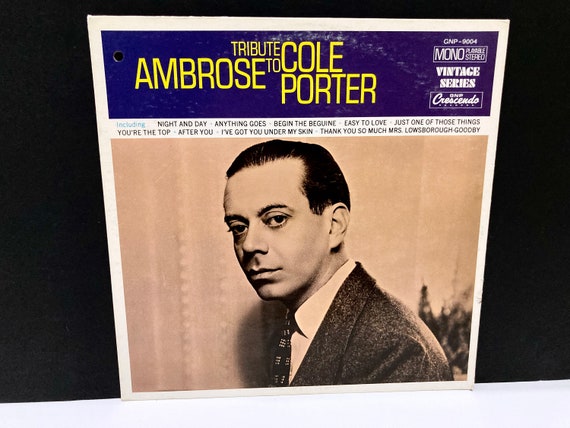The image showcases a vintage vinyl record cover in a color photograph with a black background slanted upwards to the right. The cover features a large black-and-white photograph of a man, presumably the musician or conductor, dressed in a dark suit, white undershirt, and black-and-white tie. The man, with slicked-back black hair, faces the left side of the image but turns his head to look at the viewer. Across the top is a dark blue horizontal rectangle with yellow text on the left, reading "Tribute to Ambrose Cole Porter," and white text logos on the right, including "GNP 9004," "mono," "playable stereo," and "vintage series." Under the blue rectangle are two rows of song titles in white text, listing tracks such as "Night and Day," "Anything Goes," "Begin the Beguine," "Easy to Love," "Just One of Those Things," "You're the Top," "After You," "I've Got You Under My Skin," and "Thank You So Much, Mrs. Lousborough, Goodbye." The entire design is set against a black backdrop, emphasizing the classical and timeless nature of the tribute.